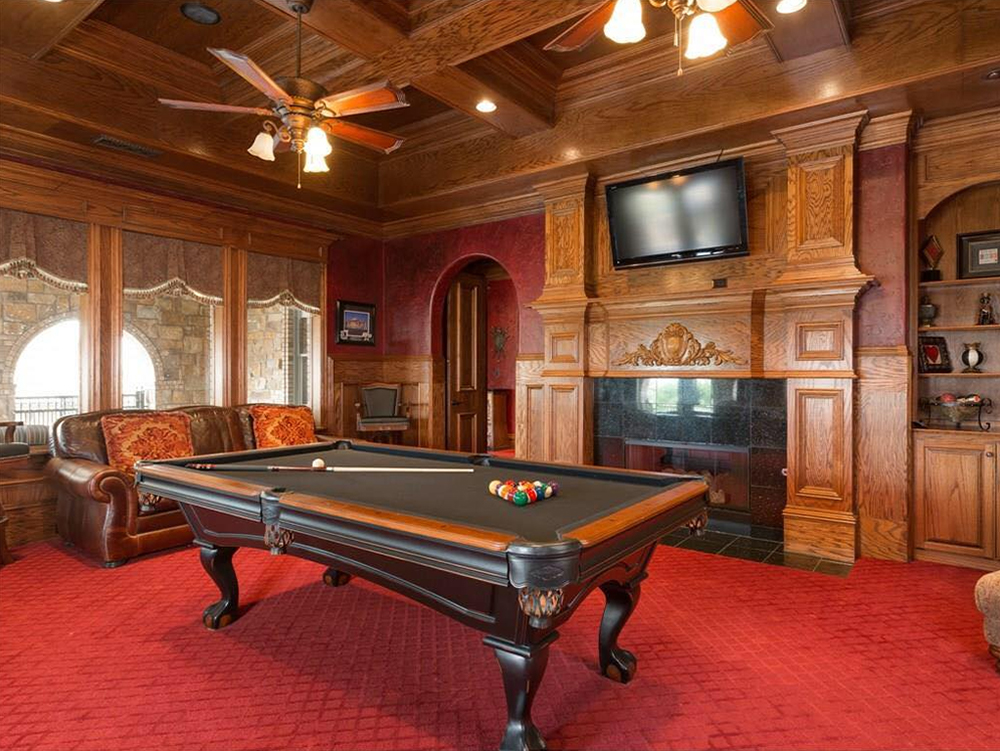The photograph depicts a luxurious billiards room within a grand, likely expensive, home or mansion. The room features rich, ornate wood paneling and built-in bookshelves adorned with various decorations, including pictures and knickknacks. The centerpiece of the room is a magnificent pool table with intricately carved cabriolet legs and a dark mahogany wood frame, trimmed in lighter wood and finished with leather accents. The pool table, set with a cue stick and pool balls, sits on a plush red carpet that adds a rich texture to the room's ambiance. 

A prominent feature of the room is the large flat screen TV mounted high on the paneled wall, just above the grand fireplace enclosed with a black screen. Above, the ceiling boasts crisscrossing beams and ceiling fans with integrated lighting, enhancing the room's grandeur. To the right of the fireplace, built-in shelving units house more decorative items, further emphasizing the room's lavish yet old-fashioned aesthetic. 

A brown leather sofa, accented with orange and beige print pillows, is positioned against a wall. Behind the sofa, large windows allow natural daylight to filter into the room, although the view outside remains obscured. A distinctive round doorway on the far left leads to another part of the house, completing this sumptuous and meticulously detailed space which epitomizes opulence and a touch of timeless elegance.